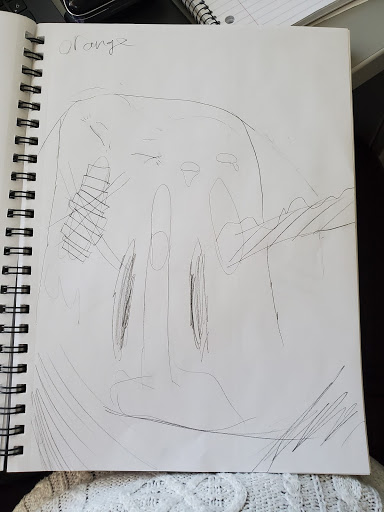A child's drawing, reminiscent of a carefree and imaginative moment, adorns the page of a spiral-bound notebook. The artwork lacks a definitive shape or form, embodying the whimsical nature of unfettered creativity. Dominating the top left corner, the word "oranges" is scrawled in a playful attempt at spelling, missing the final 'e' and replacing it with a 'z'. A figure, possibly intended to be a backpack, emerges from the chaos, roughly shaped like a rounded rectangle. The notebook’s black rings frame the left side of the page, capturing the essence of spontaneous, youthful artistry.